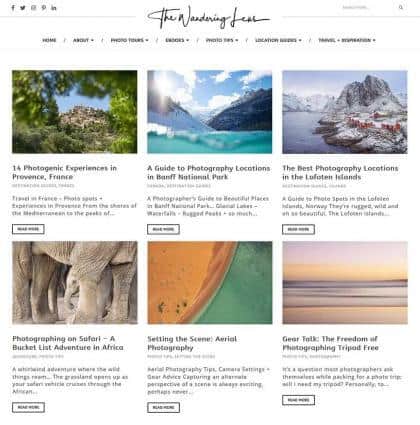This image shows the results of a search for a specific website. In the center, written in cursive, the word "wandering" is clearly visible, although the final word is obscured. The page features a grid layout with six images arranged in two rows of three. The first image presents a mesmerizing view through a tunnel of lush green leaves leading to a majestic rock mountain. Adjacent to this, the second image depicts a similar rocky formation under a pristine blue sky, with a tranquil body of water in the foreground. These images predominantly showcase breathtaking landscapes. The bottom left image deviates slightly, featuring parts of elephants, including a baby elephant, accompanied by the caption "Photographing on Safari: A Bucket List Adventure in Africa." Finally, another discernible image is a serene beach scene, capturing gentle waves rolling onto the shore.